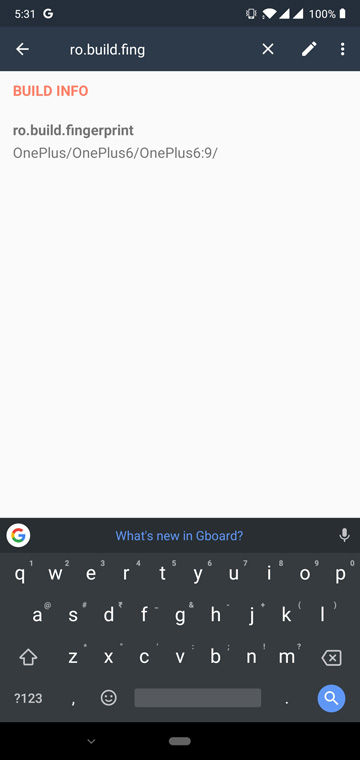This is a detailed image of a cell phone screen. At the top of the screen, against a black border, the time reads 5:31. To the right, there is a 'G' icon indicating Google, and additional status icons showing internet connection, cellular signal, and a battery icon with '100%'.

Below the time and status bar, there is a small left-pointing arrow and text that reads "go.build.fing". Accompanying this text are a white 'X' icon, a pencil icon, and an icon with three vertical dots. Underneath these elements, 'Build Info' is prominently displayed in orange text.

The majority of the screen has a very light gray background. Within this space, in orange text again, it displays "Build Info", followed by "ro.build.fingerprint: 1+ / 1+6 / 1+6:9/". 

Towards the bottom of the screen, there is a keyboard overlay with a dark gray background. In the top left corner of this overlay, there is a white circle containing the Google logo, next to blue text that reads "What's new in Gboard". In the top right, there's a microphone icon.

The virtual keyboard itself is displayed in a standard QWERTY layout. The top row shows "QWERTYUIOP", the middle row "ASDFGHJKL", and the bottom row "ZXCVBNM" along with additional keys: an upward-pointing arrow, a question mark/123 key, a comma, a smiley face icon, a space bar, a period, and a search bar. The entire screen is framed by a black border at the bottom.